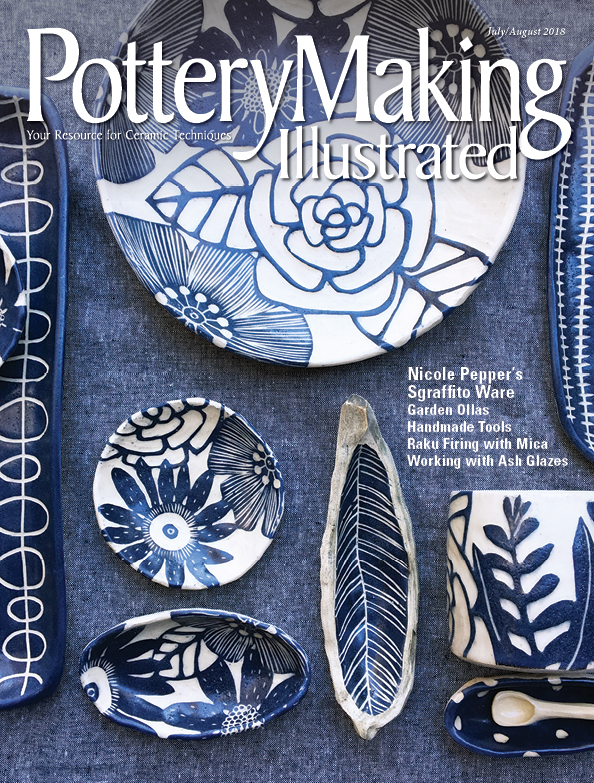This is a photograph of the cover of the July-August 2018 issue of Pottery Making Illustrated magazine. The magazine title, "Pottery Making Illustrated," is prominently displayed in large white letters at the top, with the tagline "Your Resource for Ceramic Techniques" positioned to the left. In the top right corner, the issue date is printed in small white letters. Various feature articles are highlighted on the cover, including "Nicole Pepper's Sgraffito Ware," "Handmade Tools," "Raku Firing with Mica," and "Working with Ash Glazes."

The cover image features a collection of ceramic pieces artistically arranged on a blue denim-like tablecloth, creating a visually striking display dominated by blue hues. Central to the image is a large white plate adorned with blue floral motifs, drawing the viewer's eye. Below and to the left of the large plate is a smaller matching dish, also decorated with blue flowers. Adjacent to the smaller dish is an oblong serving piece featuring a single leaf design rendered in a dark blue glaze. There is also a floral coffee cup accompanied by a blue polka dot spoon rest, and a tall, skinny ceramic piece with dark blue glaze and white circular patterns running down its length, located on the left border of the image.